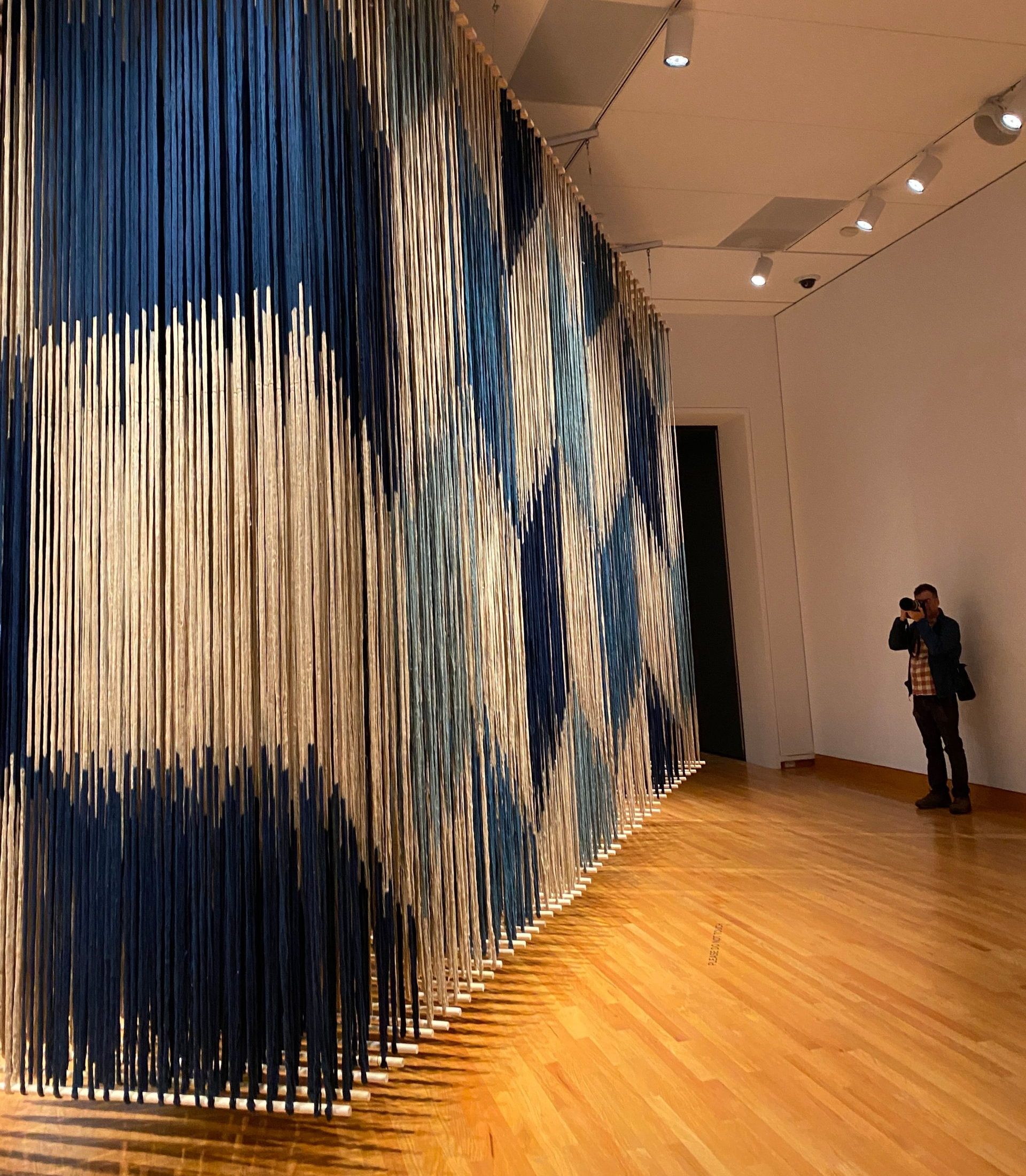The image depicts an art gallery featuring an expansive loom as the central piece of art. On the right-hand side of the image, a man stands on a wooden floor against a white wall, engrossed in photographing the artwork. He is dressed in a plaid shirt with a jacket over it, dark jeans, and boots, and his brown hair is visible. He holds a professional camera in an upright position.

The loom, dominating most of the frame, showcases a striking woven pattern in shades of dark blue, light blue, and creamy beige. Studio lights from the ceiling illuminate the art, highlighting its intricate details. Behind the loom, a black doorway is partially visible, adding depth to the scene. Wooden beams at the top and bottom of the loom indicate where the fabric is stretched, contributing to the captivating complexity of the artwork. The entire scene reflects a meticulous and creative atmosphere, emphasizing the loom's impressive craftsmanship and visual appeal.